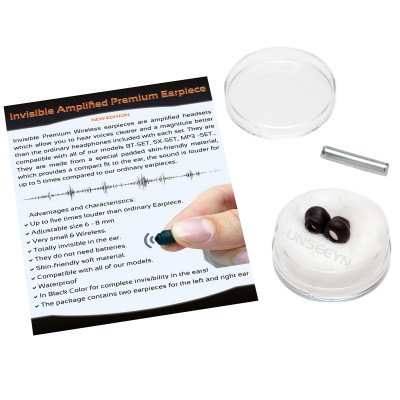The image displays the "Invisible Amplified Premium Earpiece" against a white background. Prominently featured are three objects: a white, shallow container with its lid removed, showing a small black earpiece nestled inside. Beside the container, a finger and thumb delicately hold another identical earpiece, emphasizing its compact size. To the left of these objects, a nearly square card provides detailed information about the earpiece. The card includes a title in orange text, "Invisible Amplified Premium Earpiece," along with a paragraph of descriptive text and approximately 12 bullet points outlining features such as waterproofing, being totally invisible when worn, and offering sound amplification five times greater than ordinary earpieces. The entire setup is arranged horizontally, highlighting the earpiece's innovative design and functionality.